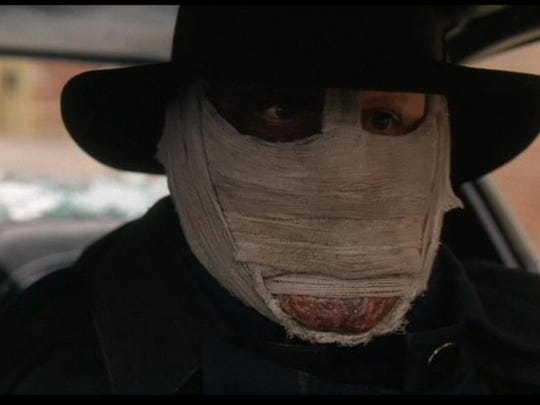A close-up image shows a man sitting in the front seat of a car, with the vehicle's side and rear windows visible around him. His face is extensively wrapped in white, slightly discolored bandages, leaving only his eyes and a small portion of his chin exposed. The bandages, which may signify an injury, cover his entire face except for these eye and chin areas. The man's skin appears discolored with a mix of burned and normal skin tones. He is wearing a large-brimmed black hat, sunglasses, and a heavy black trench coat with a collar. His chin, exposed through the bandages, shows signs of possible disfigurement, adding to the overall impression of a severe injury or medical condition.